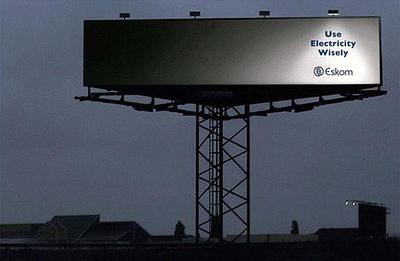This image captures a nighttime scene featuring a prominent billboard elevated on a metallic structure. The sky is a dim, dark gray, indicating it is either dusk or early night. The billboard itself is long and rectangular with a gradient background shifting from black on the left to white on the right. It is illuminated by four lights mounted on top, though only the rightmost light is functioning, casting a spotlight on the words "Use Electricity Wisely." These words are displayed in a dark font and occupy the central part of the billboard. Beneath this slogan, in smaller text, is the name "ESKOM" accompanied by a circular logo on the bottom right corner. Silhouetted houses and other structures, including rooftops and chimneys, are faintly visible against the gray sky, adding depth to the background. The overall ambience conveys a subtle reminder to conserve electricity.